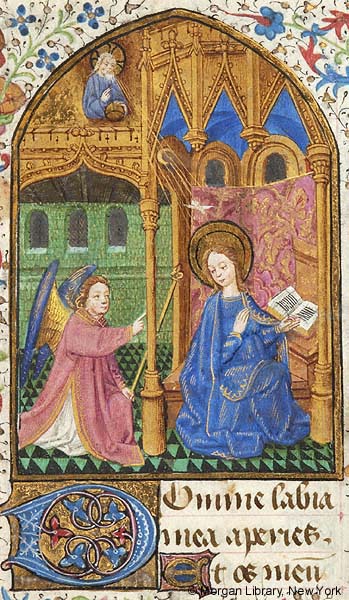This image is a highly detailed medieval artwork, likely a religious piece, that appears to be set indoors. It features several figures and vibrant colors. At the top left, there is a man who seems to be emanating light towards a woman situated on the middle right, perhaps suggesting a divine or spiritual connection. This woman, described with brown hair, is seated on a gold or bronze throne with an ornate pink and gold seat back, and she is wearing a blue robe. She is holding a book placed upon a stand.

To the middle left, there is another female figure dressed in a pink robe with a white sheet underneath, who could be a young girl. She is pointing towards the seated woman, and notably features gold and blue wings, hinting at angelic qualities. The scene is filled with colors like white, rose pink, darker green, gold, and bronze.

Additionally, there's text at the top of the image in a language that is not English, and a watermark at the bottom reads "Morgan Library, New York." Overall, this rich and colorful illustration appears to be something you might find in a museum, with a strong medieval and religious theme.